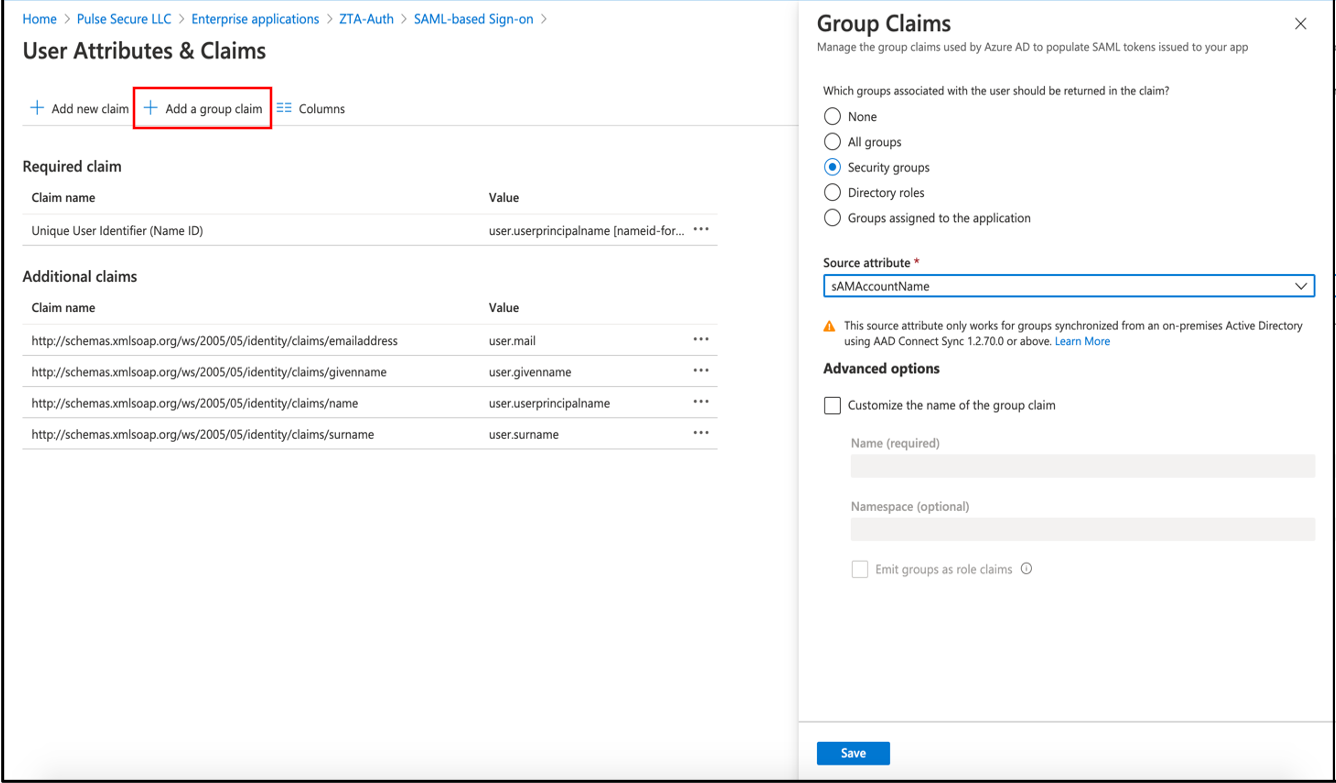Screenshot from Administrative Interface Displaying Group Claim Addition in SAML-Based Sign-On Section

The image is a screenshot of an administrative site showcasing a SAML-based sign-on section, specifically focusing on user attributes and claims management. The navigational path at the top of the page is highlighted in blue, reading: "Home > Pulse Secure LLC > Enterprise Applications > ZTA Off > SAML-based sign-on".

In the currently viewed section, there is an option to "Add new claim" and "Add a group claim", with a prominent red box surrounding the "Add a group claim" button. Below this, the term "Required claim" introduces a table with columns for "Claim name" and "Value". The "Claim name" is marked as "Unique user identifier (Name ID)" with a corresponding "Value" which consists of a long user identification string.

Further down, under the "Additional claims" section, there is another table displaying "Claim name" and "Value". This section lists several URLs under "Claim name" and their corresponding values on the right, labeled as user.mail, user.givenname, user.userprincipalname, and user.surname.

On the far right side of the screen, additional options for managing group claims are visible.

This detailed administrative interface allows users to manage claims effectively within the SAML-based sign-on framework.